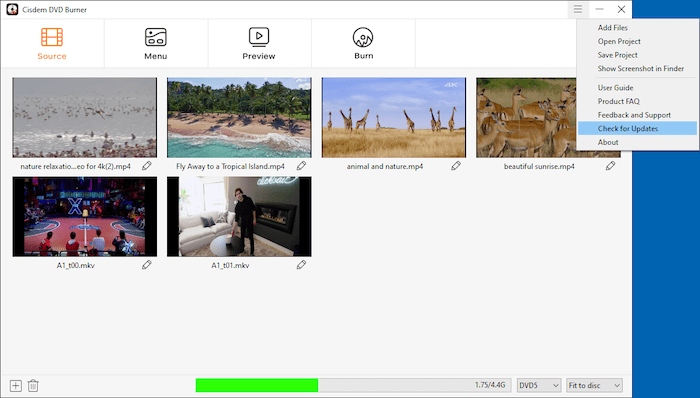The image depicts a split-screen computer interface with distinct sections and various elements. On the right side of the screen, there is a solid blue background with a gray pop-up window overlay. Adjacent to this, on a white background, located at the upper right corner, are three horizontal gray lines resembling a menu icon, followed by a single gray line, and a black 'X' icon. The three gray lines indicate an active menu, as evidenced by the gray highlight, suggesting it's been clicked.

The gray pop-up menu displays several options in black text: "Add Files," "Open Project," "Save Project," "Show Screenshot in Finder," with a dividing gray line beneath these options. Below the line, additional options include "User Guide," "Product FAQ," "Feedback and Support," and "Check for Updates," which is highlighted in blue, indicating recent selection. The menu concludes with "About."

On the left side of the screen in the white background area, labels are visible: "System," "DVD Burner," and an orange-highlighted "Source." Below these, black text denotes "Menu," "Preview," and "Burn." Under these labels are several file listings, each representing different media files, likely videos. These include:

1. "Nature Relaxation 4K.mp4"
2. "Fly Away to a Tropical Island.mp4"
3. "Animal Nature.mp4"
4. "Beautiful Sunrise.mp4"
5. "A1_T00.mkv"
6. "A1_T01.mkv" 

The detailed listings display a mix of nature-themed videos and some files labeled with technical identifiers, possibly originating from different sources or projects. The entire scene conveys a working interface for some media management or video burning software.